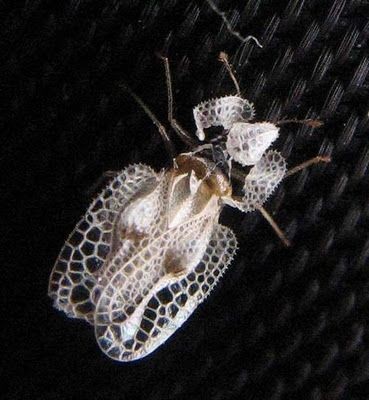The photograph captures an extreme close-up of a highly magnified insect, possibly known as a lace bug. The insect is positioned centrally on a black surface, speckled with gray pocks. Its intricate structure appears skeletal and semi-transparent, suggesting it might be an exuvia or the remains of a bug. The head features two flap-like extensions on either side and a central teardrop-shaped portion. The body is diaphanous, showcasing web-like, lattice patterns that extend into what appears to be wings. These wings are lined with delicate, skeletal veins. The creature has six thin legs, and its head and body exhibit a milky white hue with lace-like structures, enhancing its ethereal appearance.